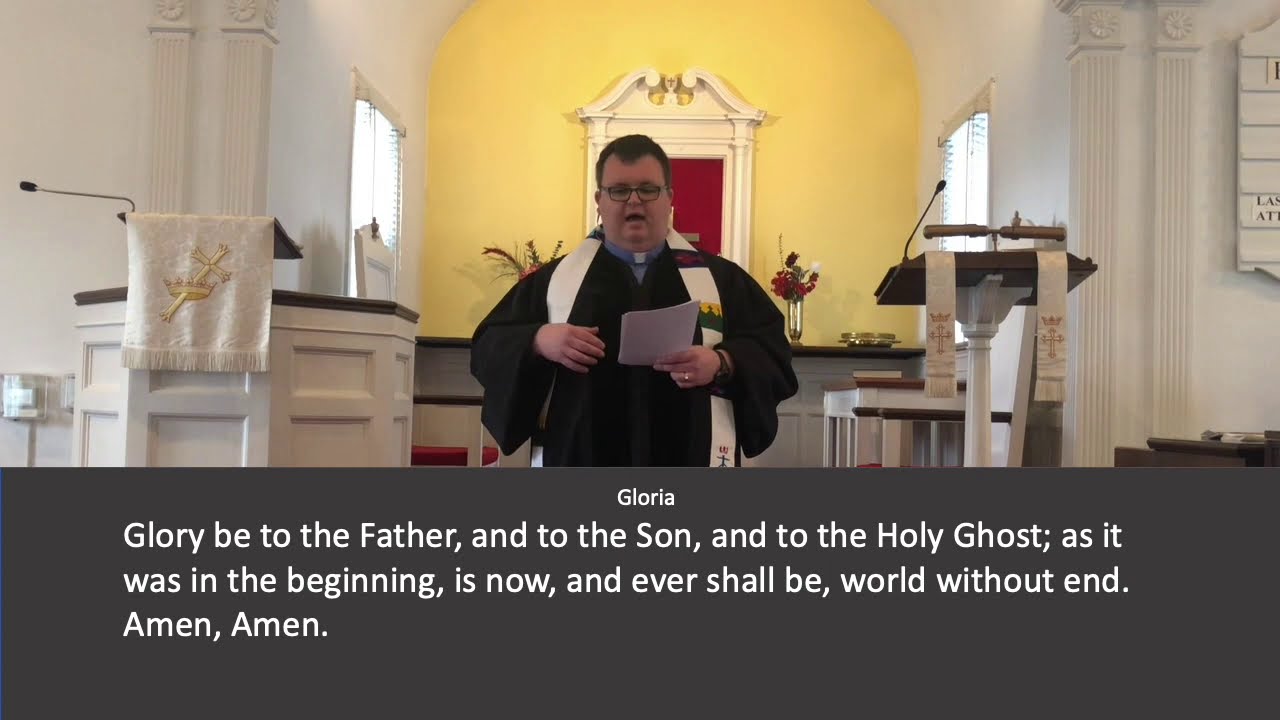In the image, a priest is seen delivering a sermon inside a church. Dressed in a black robe with a distinct white clerical collar, he wears a white scarf adorned with blue, yellow, red, and green accents. His right hand holds a sheet of paper while his left hand hovers close by, as though guiding his reading. The priest, who has receding brown hair and square plastic frame glasses, stands before a podium.

Behind him, a white-framed red door with an angelic symbol above it is visible, flanked by yellow walls. There are windows to the left and right of the door, and additional church elements such as crosses, flowers, a statue on the right, and a plant on the left can be seen. The background also includes architectural details like pedestals and parts of the wall.

Beneath the priest, occupying the lower portion of the image, is a dark gray rectangular box displaying text in white. At the center-top of this box, the word "Gloria" appears, followed by the text: "Glory be to the Father, and to the Son, and to the Holy Ghost, as it was in the beginning, is now, and ever shall be, world without end. Amen, amen."